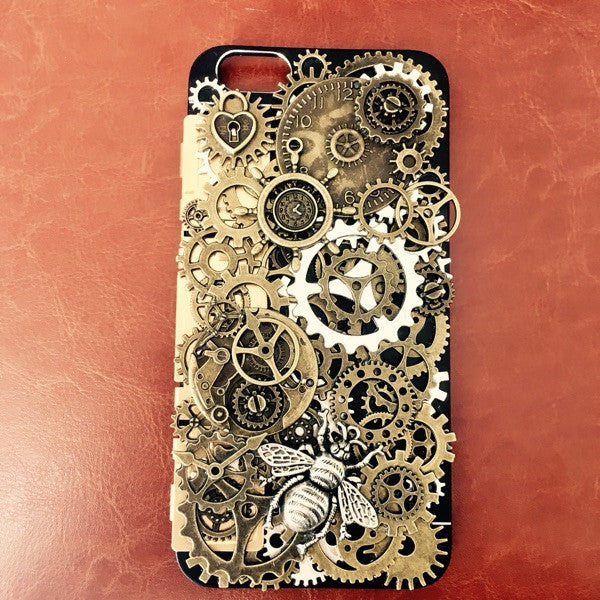This image is a detailed photograph of a black iPhone case, specifically designed for an iPhone X or earlier models with a single camera. The case is adorned with an intricate arrangement of metal gears and watch parts, predominantly in gold and brassy copper tones. These gears, varying in size and design, cover the entire surface of the case. Notable features include a clock face near the camera and a heart-shaped locket integrated within the gears. Additionally, a large gold, metallic bee charm is prominently attached near the bottom center of the case, looking diagonally upward towards the top right of the image. The background of the photograph is a distressed, reddish-brown leather material, adding a textured backdrop that enhances the detailed elements of the phone case.